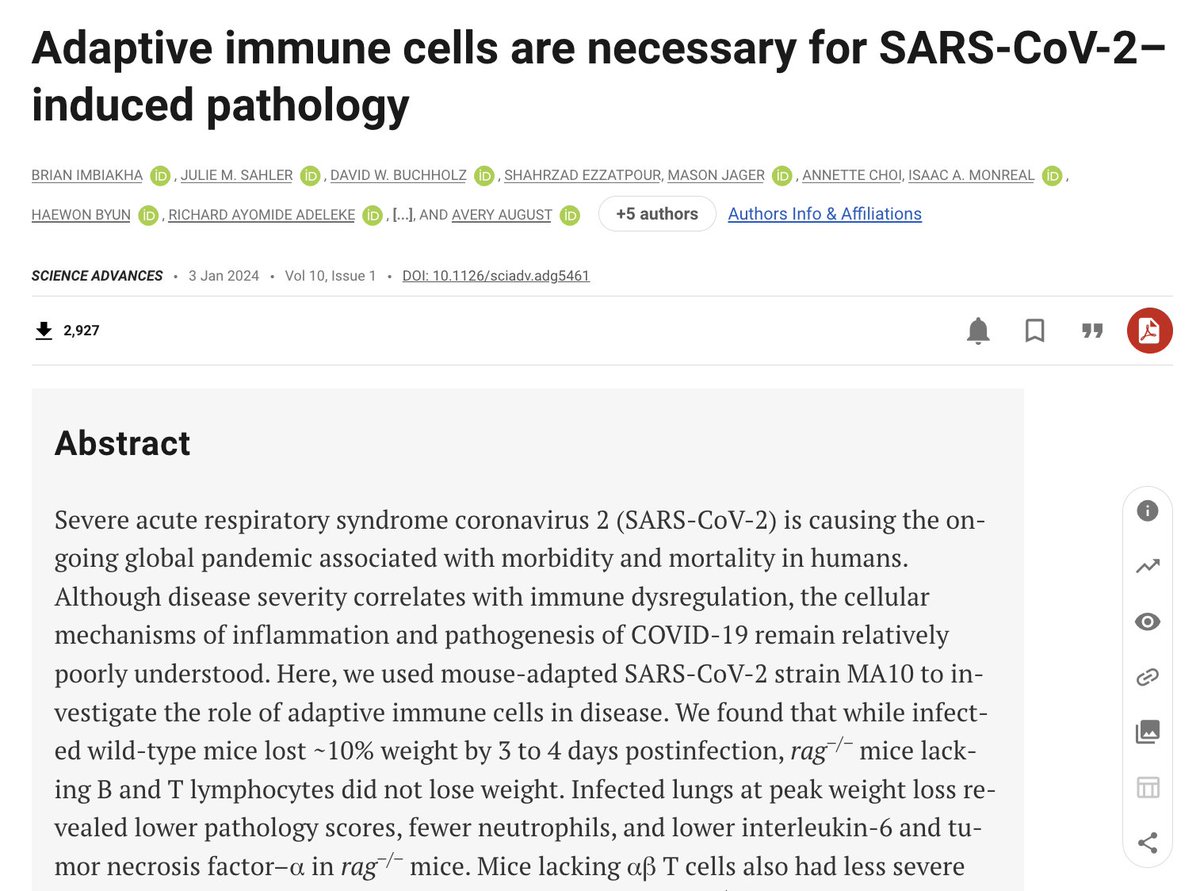This is a website screenshot featuring an article from Science Advances, titled "Adaptive Immune Cells Are Necessary for SARS-CoV-2-Induced Pathology." The article, published in Volume 10, Issue 1 on January 3, 2024, lists a total of 13 authors, although their affiliations are not provided. The article has been downloaded 2,927 times and includes an abstract that reads:

"Severe acute respiratory syndrome coronavirus 2 (SARS-CoV-2) is causing an ongoing global pandemic associated with significant morbidity and mortality in humans. Despite the correlation between disease severity and immune dysregulation, the cellular mechanisms driving the inflammation and pathogenesis of COVID-19 remain relatively poorly understood. In this study, we used a mouse-adapted SARS-CoV-2 strain (MA10) to investigate the role of adaptive immune cells in disease progression. We discovered that while infected wild-type mice lost 10% of their body weight within three days post-infection, RAG-deficient mice, which lack functioning B and T lymphocytes, did not exhibit weight loss. Furthermore, infected lungs at the peak of weight loss in wild-type mice showed higher pathology scores, increased neutrophil infiltration, and elevated levels of interleukin-6 and tumor necrosis factor. In contrast, RAG-deficient mice exhibited lower pathology scores and less severe inflammatory responses."

The article offers crucial insights into the role of adaptive immune cells in the pathology of SARS-CoV-2, emphasizing the significance of these cells in mediating the disease's inflammatory response.